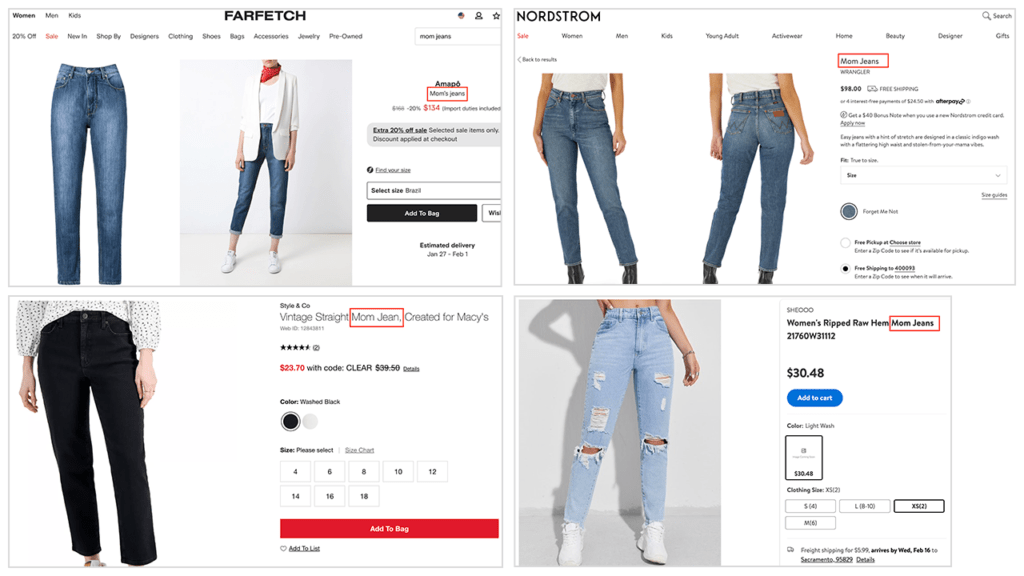The image is a collage of four different screenshots, each from various websites showcasing blue jeans for sale.

- **Top Left:** The website displayed is Farfetch, as indicated by the 'Farfetch' label at the very top center. Below it, there is a navigation bar with several clickable text tabs leading to different web pages. The main content features two images of a pair of blue jeans: one front-view and another worn by a model. On the right, there is some textual information which is too blurred to decipher.

- **Top Right:** This section is from the Nordstrom website, with 'Nordstrom' written in the top left corner. The featured product is also blue jeans, displayed in two images showing front and back views on a model.

- **Bottom Left:** Here, a pair of black jeans are showcased on a model. A prominent red text box with the words "mom jeans" is highlighted in the description across all images.

- **Bottom Right:** This portion displays a single image of blue jeans with ripped details worn by a model. The price is prominently shown as $30.48.

Each section focuses on different styles and details of jeans, presented on models to highlight their fit and appearance.